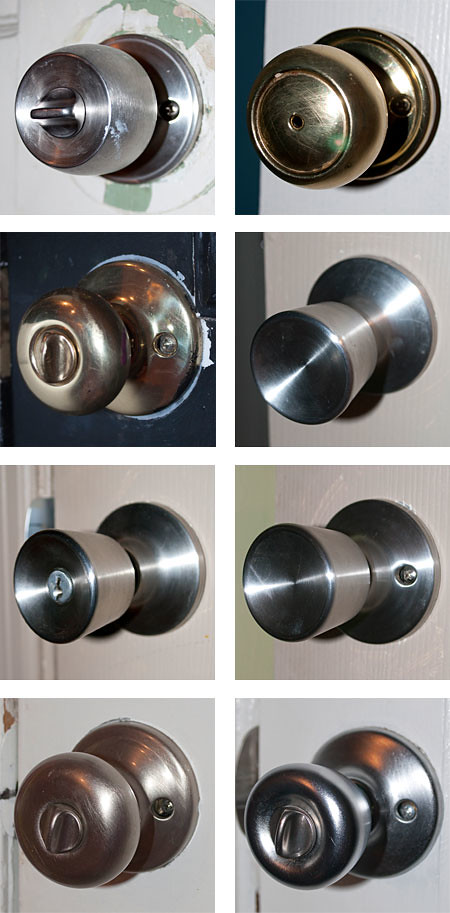The image showcases a grid of eight distinct doorknobs, arranged in two columns of four, creating a symmetrical layout with a small gap between each square, forming a clean white grid pattern. Each doorknob is centered within the square and varies in color and design. The top left doorknob is silver with a small turn lock in the middle, followed by a gold rounded knob below it, also featuring a turn lock. The third doorknob down on the left is a silver exterior knob with a locking mechanism, while the bottom left displays a gold rounded knob with a turn lock. On the right side, the top knob is gold with a keyhole, and directly beneath it is a silver knob with no visible lock or keyhole, but differentiated by the presence of a screw on the third knob down. The bottom right doorknob is silver, rounded, and equipped with a turn lock. The overall background is gray, enhancing the contrast between the doorknobs and ensuring each one stands out clearly.